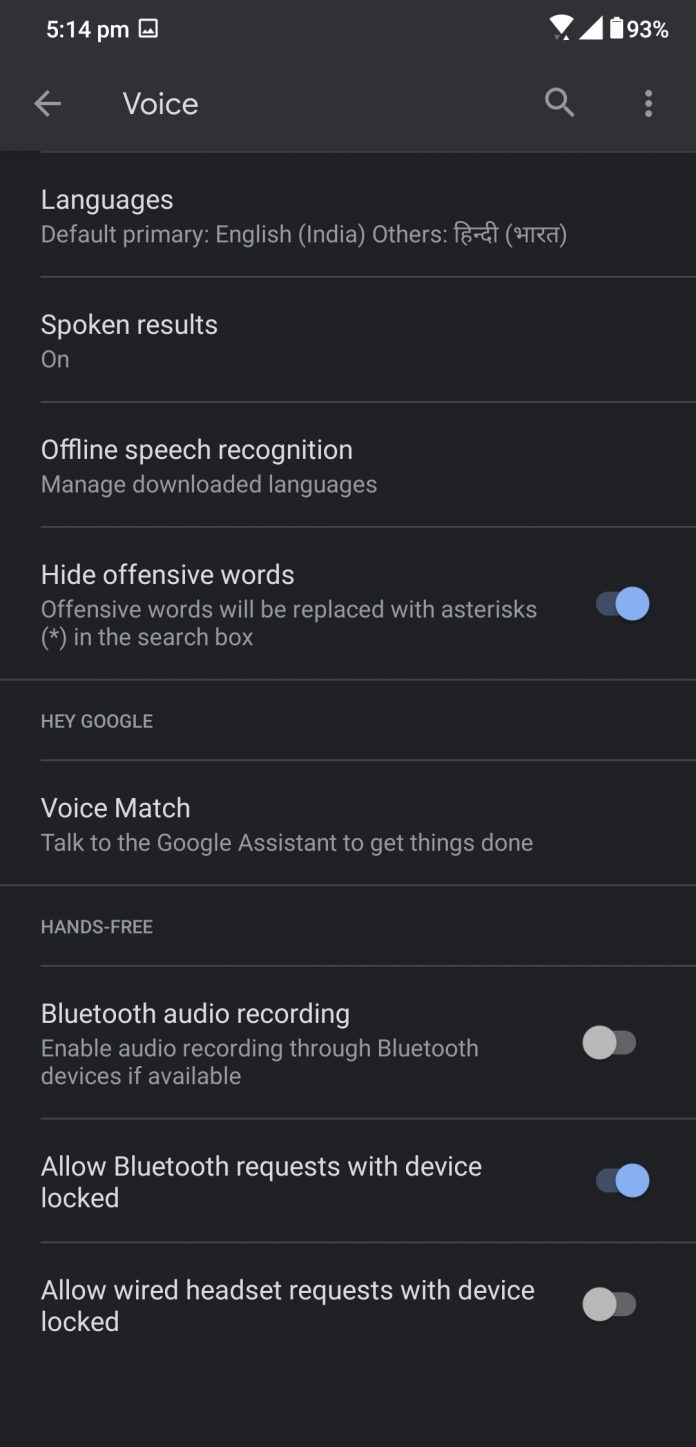The image displays a detailed settings page on a mobile phone, likely related to voice control or Google Assistant settings. 

1. **Status Bar**:
   - **Time**: 5:14 PM displayed on the top-left.
   - **Icons**: Next to the time, there is a square icon with dots whose purpose is unclear.
   - **Connectivity Status**:
     - Wi-Fi indicator (active/connected).
     - Cell service indicator (full strength).
   - **Battery**: A battery icon showing a high charge level beside "93%".

2. **Search Bar**:
   - **Text**: "voice" in grey letters followed by a leftward-facing arrow.
   - **Icons**: On the right, there is a magnifying glass and three vertical dots indicating settings or options.

3. **Settings Sections**:
   - **Languages**:
     - Title in bold: "Languages".
     - Details: "Default primary: English (India)" followed by other languages in foreign text.
   - **Spoken Results**:
     - Title in bold: "Spoken results".
     - Status: "On".
   - **Offline Speech Recognition**:
     - Title in bold: "Offline speech recognition".
     - Action: "Manage downloaded languages".
   - **Hide Offensive Words**:
     - Title in bold: "Hide offensive words".
     - Description: "Offensive words will be replaced with asterisks (*)."
     - Toggle: Blue sliding button indicating it is turned on.
   - **Hey Google**:
     - Title: "Hey Google".
   - **Voice Match**:
     - Title in bold: "Voice match".
     - Description: "Talk to the Google Assistant to get things done".
   - **Hands-free**:
     - Title: "Hands free".
   - **Bluetooth Audio Recording**:
     - Title in bold: "Bluetooth audio recording".
     - Description: "Enable audio recording through Bluetooth devices if available".
     - Toggle: Grey sliding button indicating it is turned off.
   - **Allow Bluetooth Requests with Device Locked**:
     - Title in bold: "Allow Bluetooth requests with device locked".
     - Toggle: Blue sliding button indicating it is turned on.
   - **Allow Wired Headset Requests with Device Locked**:
     - Title: "Allow wired headset requests with device locked".
     - Toggle: White sliding button indicating it is turned off.

Each section is separated by horizontal lines, clearly partitioning the different categories of voice-related settings.